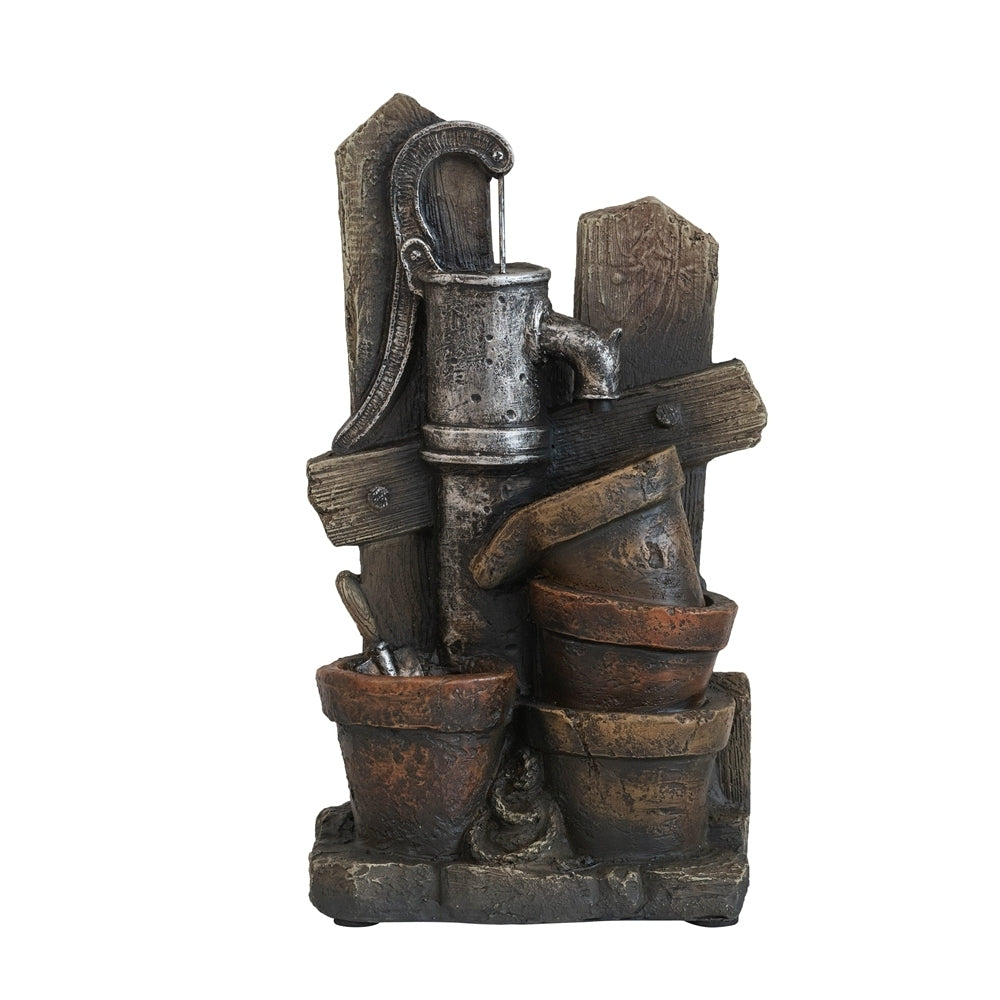The photograph depicts a rustic sculpture showcasing a vintage, manual water pump positioned against a wooden plank backdrop. The water pump, with its silvery-grey metallic sheen, stands prominently as the centerpiece. Emanating an aged and weathered charm, the entire setup includes four gardening pots—three to the right of the pump and one to the left—arranged in the foreground. These pots, in hues of dirty red and dark orange, are interconnected by a small rope, enhancing the rustic appeal. One of the pots contains a small shovel, hinting at a gardening theme. The wooden planks forming the backdrop resemble a fence, and the entire scene appears dust-covered and antiqued, giving it a sense of historical authenticity.